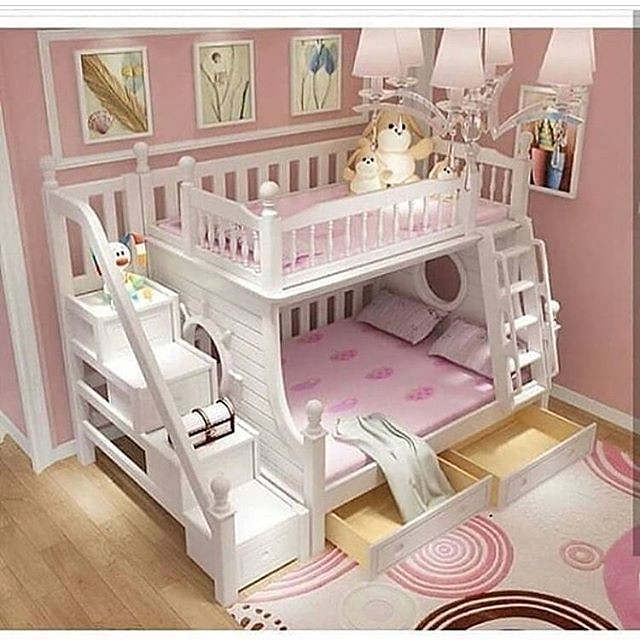The image depicts a child's bedroom, possibly from a dollhouse or a meticulously designed room display. The room has vibrant pink walls and features a bunk bed made of white wood. The bunk bed showcases a nautical theme, with circular portholes at the head and foot of the bed, as well as a ship's wheel motif on one side. The top bunk is smaller, resembling a toddler’s bed or a day bed, while the bottom bunk appears slightly wider, potentially a full-size bed, both adorned with pink sheets and pillows. Wooden stairs with railings ascend to the top bunk, and there is also a white ladder on the side near the wall. Below the lower bunk, two open drawers painted white on the outside reveal their wooden interiors. The room's floor is a light wood, topped with a white rug decorated with yellow and brown swirls. A delicate crystal chandelier with pink shades hangs from the ceiling. The walls are decorated with framed pictures, with three paintings of leaves and flowers above the bed, and a partially obstructed framed photo on the right side. Scattered around the room are stuffed animals and children’s toys, adding to the whimsical and cozy atmosphere.